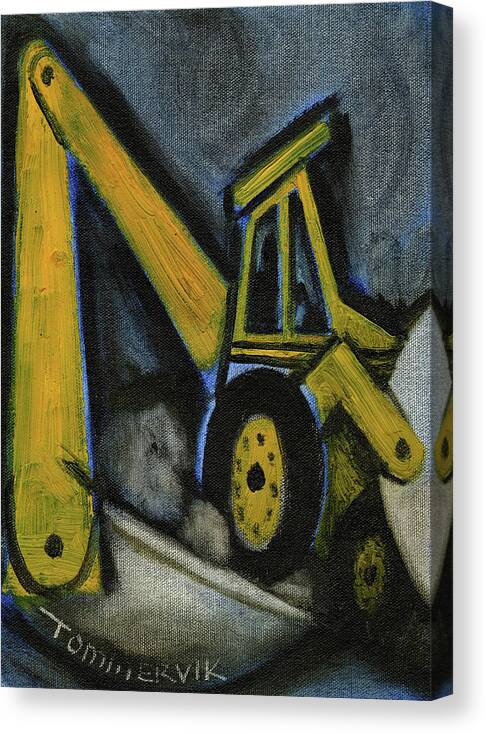The painting is a detailed, abstract depiction of a yellow tractor-like construction vehicle with an excavator-style arm. It features the artist's signature, which appears as 'Tomarvik,' curving around the bottom of the image. The vehicle, with large black tires accented with yellow, appears to be gripping a large white object in the bottom right corner. The background is a swirl of blues, grays, and whites, creating a somewhat chaotic and compressed scene. This evokes a sense of two overlapping actions that are hard to distinguish clearly. The artwork is stylized and almost three-dimensional, giving an impression of elements extending out of the canvas. Despite its complex layout, the painting captures the industrial essence of the machine, set against a moody, abstract backdrop.